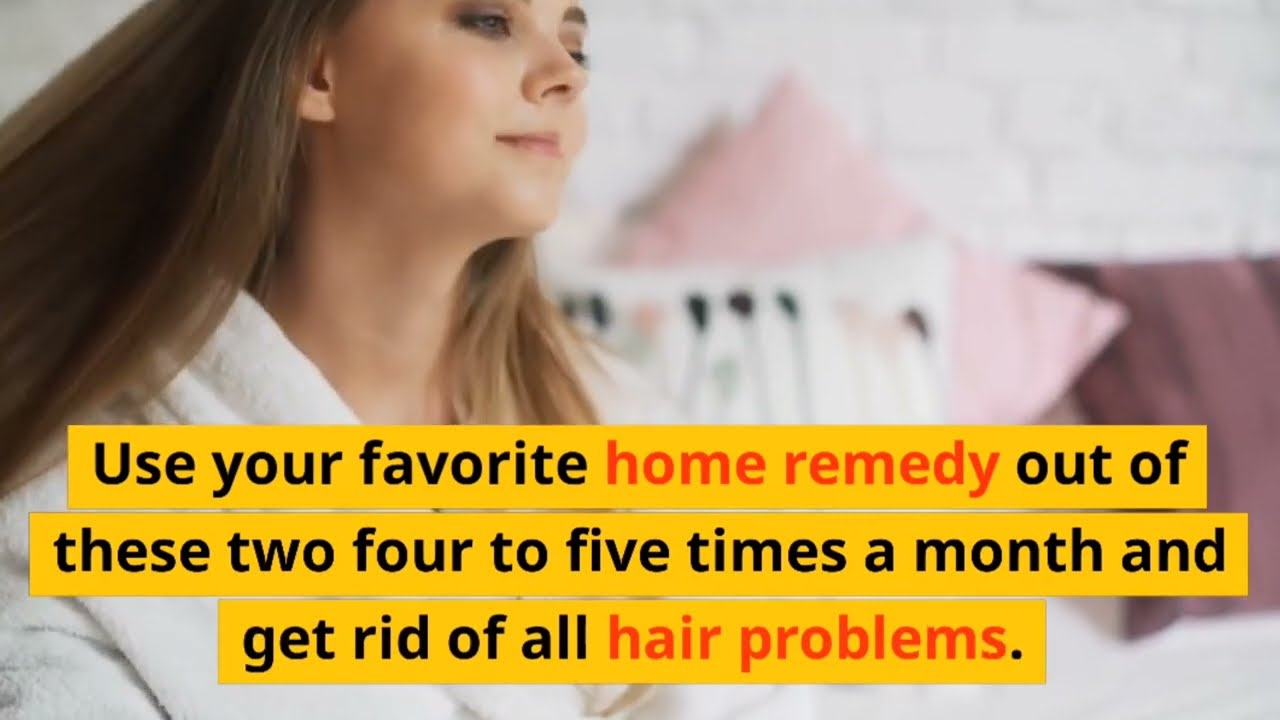The image is an advertisement featuring a young Caucasian woman positioned on the left side, shown from her eyes down to about mid-chest level. Her long, medium to light brown hair flows behind her, suggesting movement either from walking quickly or a breeze. She wears a white, fuzzy bathrobe and light brown eyeshadow. Her face is slightly tilted to the right, and her mouth is closed. The background features a blurry white brick wall with various decorative pillows in shades of pink and lavender. A yellow banner occupies about 40% of the lower part of the image, featuring black and red text that reads, "Use your favorite home remedy out of these two, four to five times a month and get rid of all hair problems."